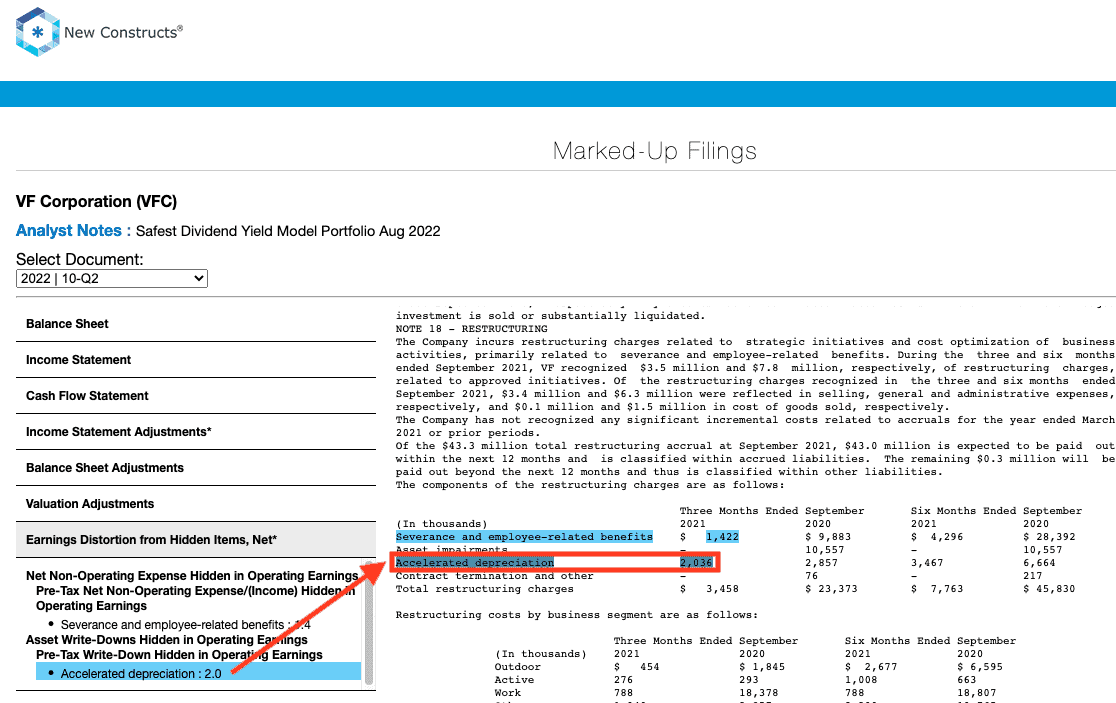Screenshot of New Constructs Interface:

The screenshot exhibits the user interface of New Constructs with a focus on financial data and analysis tools. On the left side of the screen, there is an icon composed of light blue, gray, and brown hues. Below this, a sizeable blue bar spans the width of the screen, prominently displaying the text "Marked-Up Filings." A thin gray line demarcates this section from the content below.

In the main section, there is a detailed list for VF Corporation (ticker symbol: VFC). Under "Analyst Notes," the heading "Safest Dividend Yield Model Portfolio - August 2022" is highlighted in blue. Directly beneath, there is a section labeled "Select Documents," where users can interact with various document links; one is specifically highlighted as "2022/10-QT."

Further down, the document lists multiple financial statements and adjustments:

- Balance Sheet
- Income Statement
- Cash Flow Statement
- Income Statement Adjustments
- Balance Sheet Adjustments
- Valuation Adjustments
- Earnings Distortion from Hidden Items (marked with a star)

Key details under these sections include:

- "Net Non-Operating Expense Hidden in Operating Earnings"
- "Pre-Tax Net Non-Operating Expense that is Income Hidden Operating Earnings"
- "Asset Write Downs Hidden in Operating Earnings," which is indicated as being related to accelerated depreciation, suggesting a method for reducing tax liabilities.

This screenshot captures the comprehensive financial analysis and detailed adjustments made available for evaluating the company’s performance.